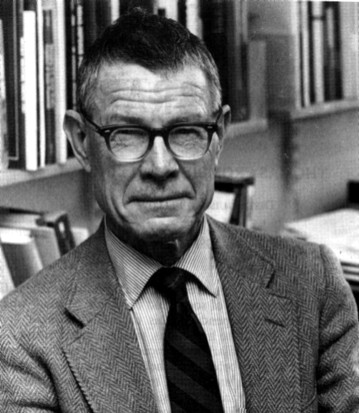The black-and-white photograph features an older, professorial-looking man seated at the center of the frame. He appears to be in his late 60s or early 70s, characterized by his wrinkled forehead, sagging cheeks, and a solemn facial expression. The man is wearing black, plastic-rimmed glasses that are dark on the top and clear on the bottom, a suit jacket that appears gray (though the image's monochrome nature makes it hard to confirm), a dark tie, and a checkered shirt underneath. His short, crew-cut hairstyle and slightly smirking mouth add to his distinguished appearance.

The background reveals a two-tiered bookshelf filled with various books. The upper level is densely packed with books, while the lower level has a more scattered arrangement with an open area to the right. The overall setting suggests an indoor environment, likely a library or an office, adding to the image’s academic ambiance. The scene is devoid of any visible text, further focusing the viewer's attention on the man and his learned surroundings. The photograph seems to date back to the late 1950s to 1970s, based on the style of the man's attire and the overall aesthetic of the image.